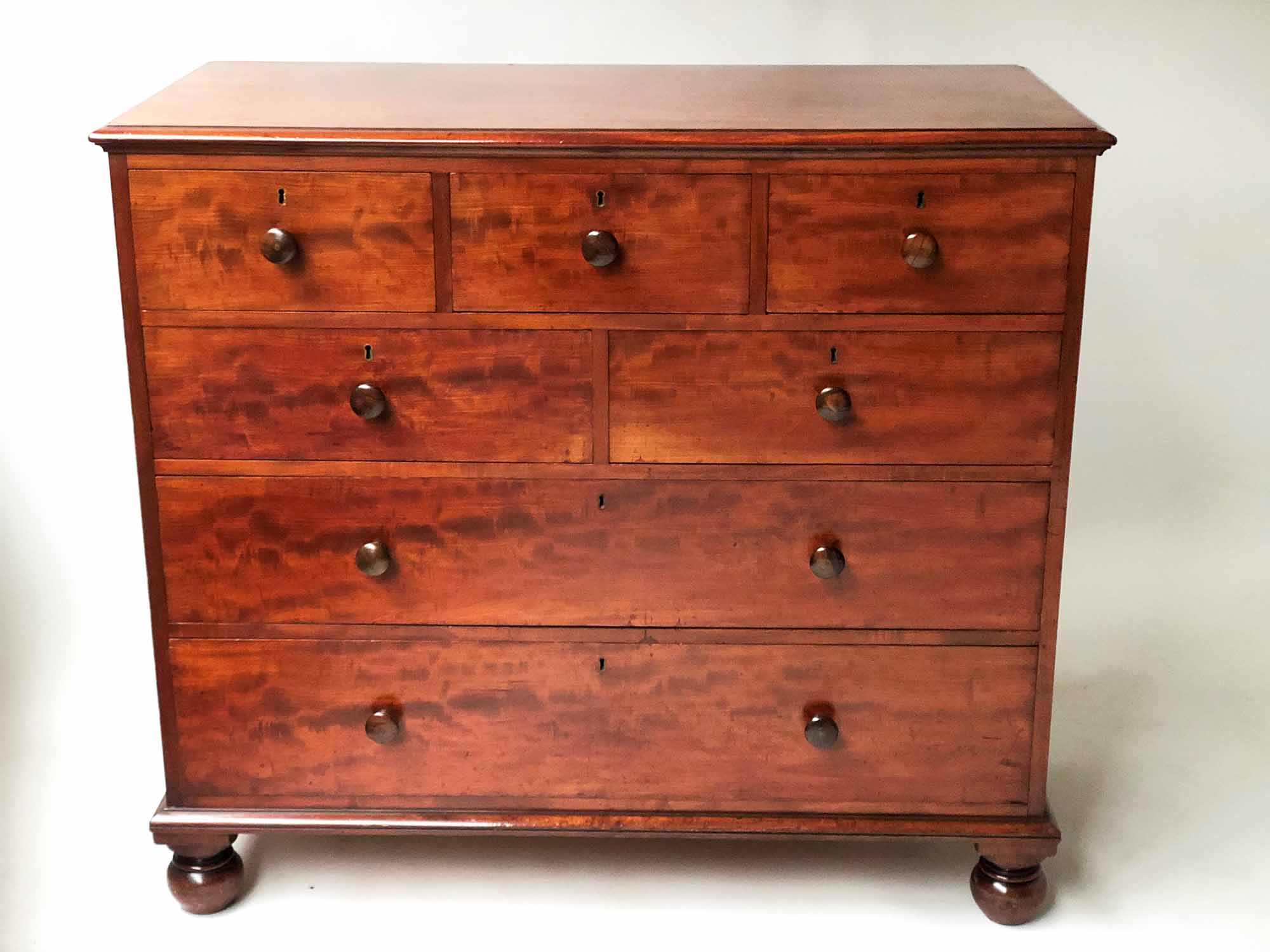The image depicts a vintage dresser made of a warm, reddish-brown wood, possibly mahogany, exhibiting a polished and glossy finish. It stands on short, spherical legs that have a reflective quality. The dresser features four layers of drawers. On the top row, there are three drawers, each equipped with a glossy knob and a keyhole above it. Below, the second row consists of two drawers, each also with a knob and corresponding keyhole. The bottom two layers each contain a single drawer, both fitted with two knobs spaced apart and a central keyhole above each. The dresser is placed against a plain white wall, reflecting its old-world charm and simplicity. Despite the image being pixelated and slightly distorted, likely for an online marketplace listing, the rich texture and smooth surface of the dresser are evident.